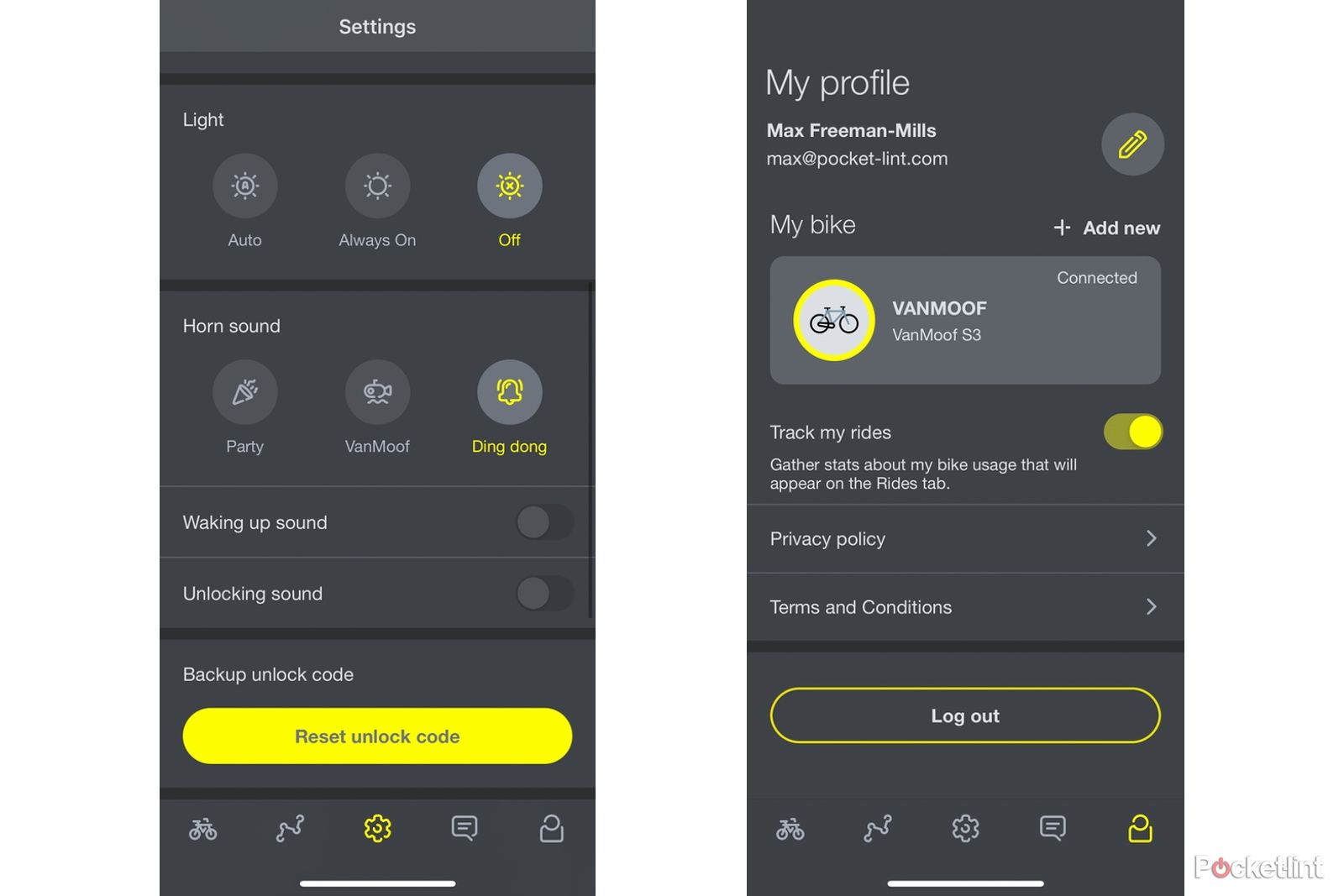The image consists of two screenshots showcasing app settings. The left screenshot displays various settings options, including:
- "Light" with three buttons: "Auto," "Always On," and "Off."
- "Horn Sound" with options: "Party," "Fan Move," and "Ding Dong."
- Settings for "Waking Up Sound" and "Unlocking Sound."
- A section for a "Backup Unlock Code" with a yellow button labeled "Reset Unlock Code."

The right screenshot highlights a user profile, with details including:
- User's name: "Max Freeman Mills"
- Email: "max@pocket-lint.com"
- Listed bike: "Fan Move S3," indicated as "Connected."
Other options available in this screenshot are:
- "Track My Rides"
- "Privacy Policy"
- "Terms and Conditions"
- A button at the bottom labeled "Log Out."